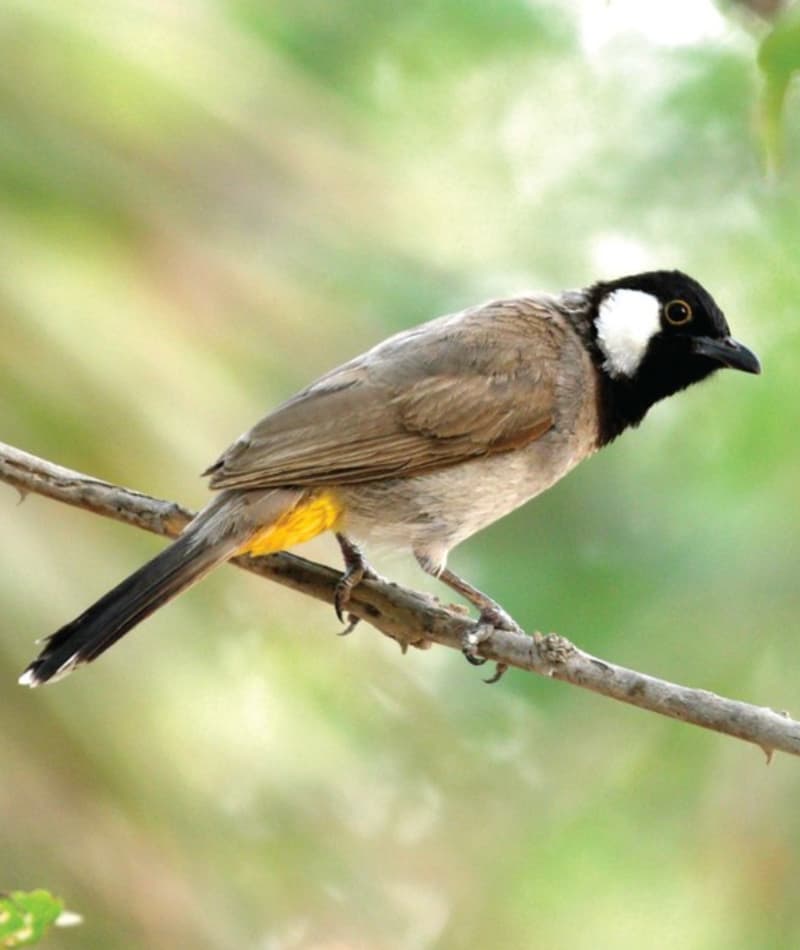The photograph captures a bird perched on a slender, bare branch that extends from the upper left to the lower right part of the image. The bird, which is primarily brown, has distinctive black feathers on its head and displays a white patch behind its black eye. Its beak is black, and beneath its legs, a patch of yellow feathers is noticeable. The tail feathers are black with white tips, with the bird’s tail positioned towards the bottom left of the frame while its head faces the right. The background is blurred, presenting an out-of-focus blend of greens, whites, and browns, hinting at trees and foliage with sunlight filtering through, suggesting an outdoor, forest-like environment. The bird's thin, clawed legs grip the branch securely, adding to the serene, natural composition of the photograph.